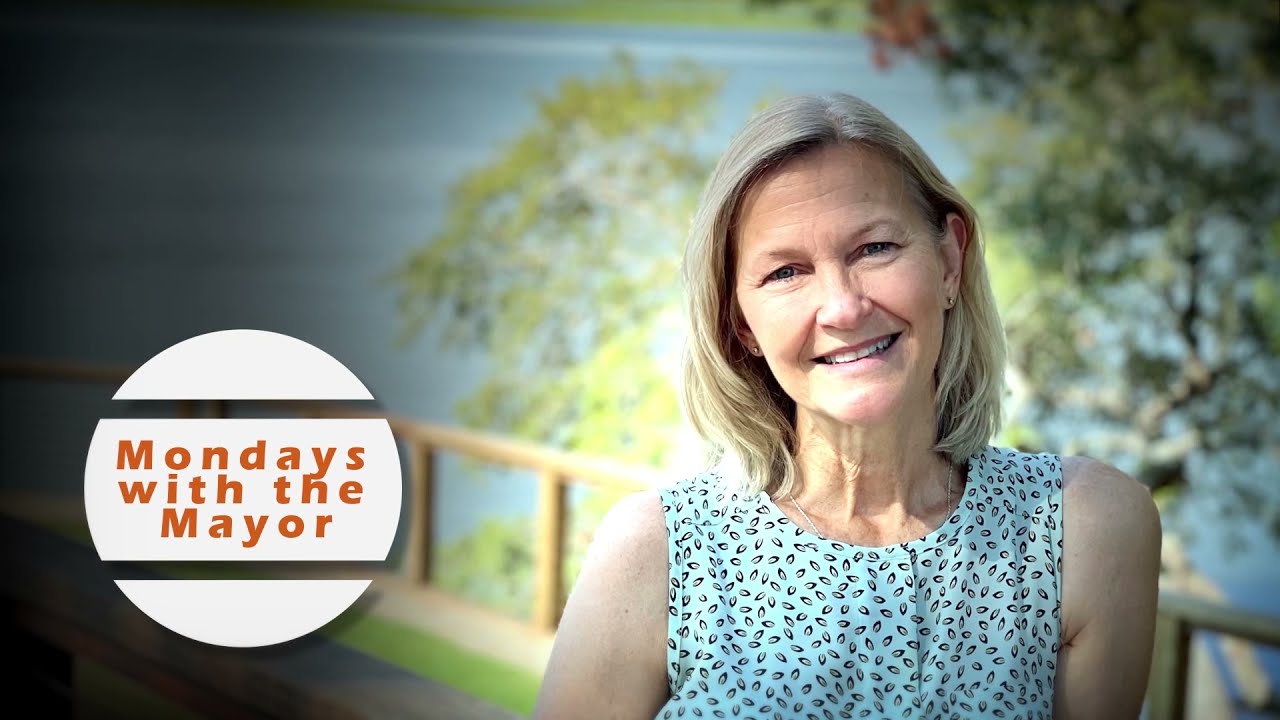The image is a daytime advertisement featuring a slightly older woman, likely in her early 50s, with a light complexion and short, light blonde hair parted in the middle. She is smiling directly at the camera, her head tilted slightly. She is dressed in a sleeveless, light blue tank top adorned with small black and white designs resembling seeds.

The background of the image is slightly blurred, showcasing a serene, blue lake and lush green trees with some gaps in the foliage. A light brown wooden fence borders the area, giving the impression she might be standing near a dock or parking lot adjacent to the lake.

On the left-hand side of the image, there is a prominent white circle with two horizontal bars, one near the top and one near the bottom, framing the text inside. The orange text within the circle reads "Mondays with the Mayor." The overall setting is well-lit with an abundance of natural light, highlighting details in the composition.